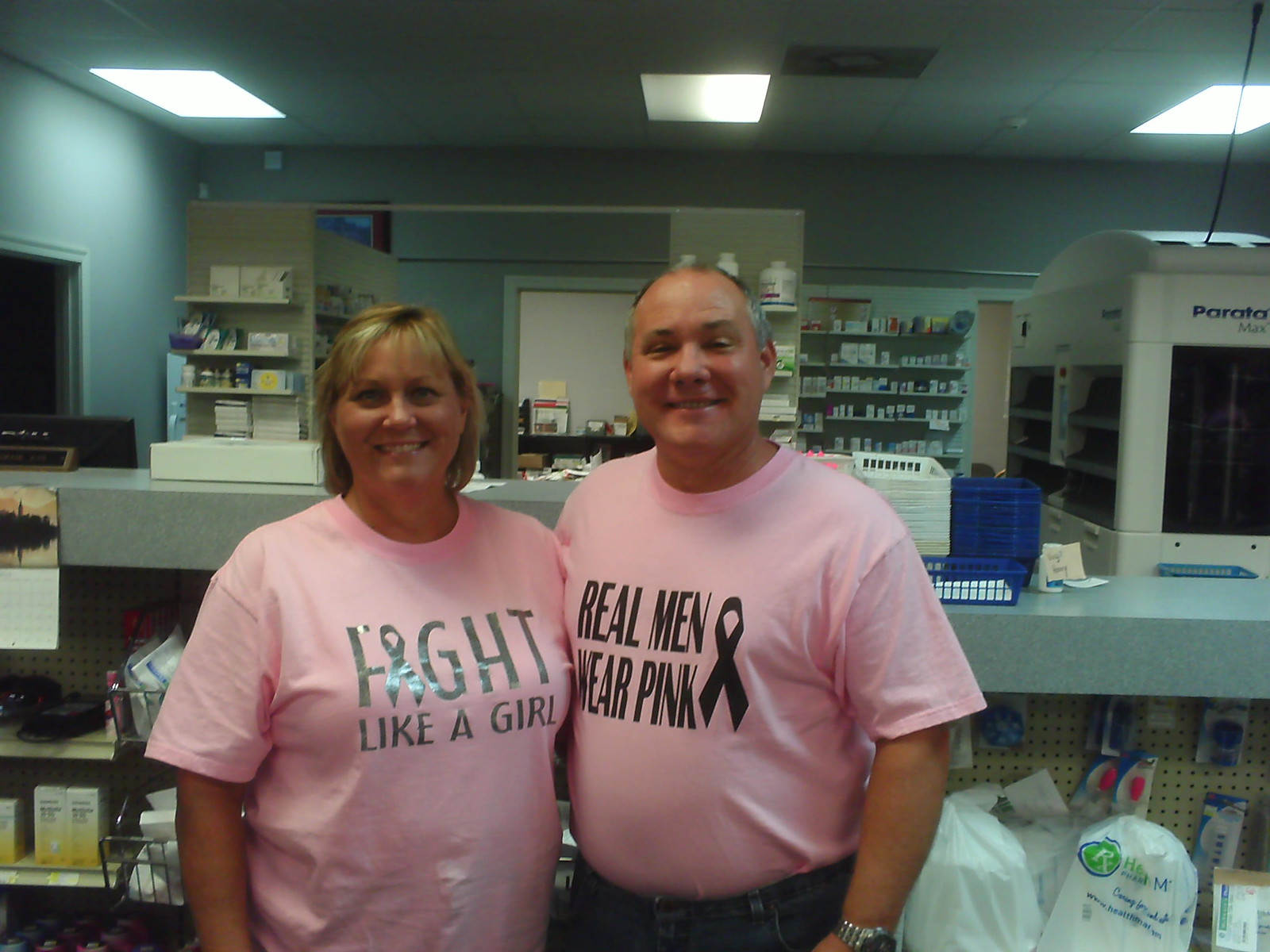In the center of a vertical rectangular photograph, a man and a woman, likely an older couple, stand proudly behind a counter in what appears to be their pharmacy. They are both wearing pink t-shirts from a breast cancer awareness campaign; the man's shirt reads "Real Men Wear Pink" with a ribbon symbol, while the woman's shirt says "Fight Like a Girl" with a ribbon forming the letter 'i' in 'Fight.' The man, positioned to the right, has dark hair with gray streaks, receding at the front, and is wearing his shirt tucked into his pants along with a wristwatch. The woman, to the left, has short blonde hair, likely dyed from brown, and is smiling. Behind them, shelves stocked with various medicine boxes and bottles line the background, indicating the nature of their business. Additional medical supplies can be seen under the counter, emphasizing the setting's professional and caregiving atmosphere.